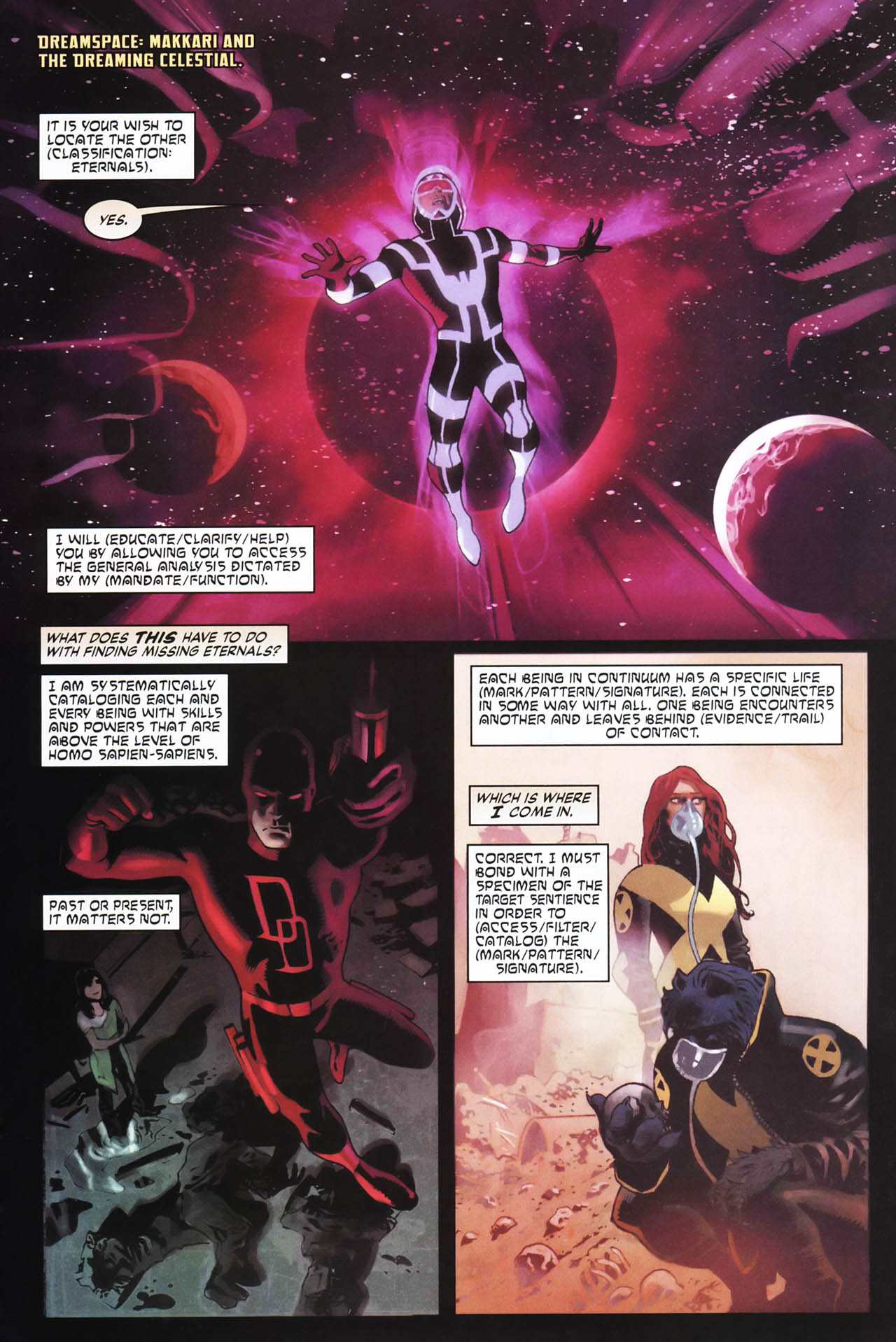This detailed comic book page features three distinct panels. The largest panel at the top is set in outer space, with a predominantly black background. Within this celestial scene, you can observe planets—one primarily in black surrounded by smaller pinkish planets. On the top left of this panel, the text reads, "Space Dream, Markkari, and Dreaming Celestial." A superhero, glowing with a pink aura and dressed in a black and white skin-tight outfit, floats prominently in front of the planets. Below this outer space scene, a speech bubble reads, "It is your wish to locate the other (Classification Eternals)." The second panel on the lower left showcases the superhero Daredevil in his signature red costume, leaping over fallen creatures in a dimly lit room. The final panel on the lower right features two X-Men characters: a woman with long red hair and Beast, depicted as an anthropomorphic blue wolfman. This composition of panels suggests a dramatic and action-filled storyline typical of Marvel comics.